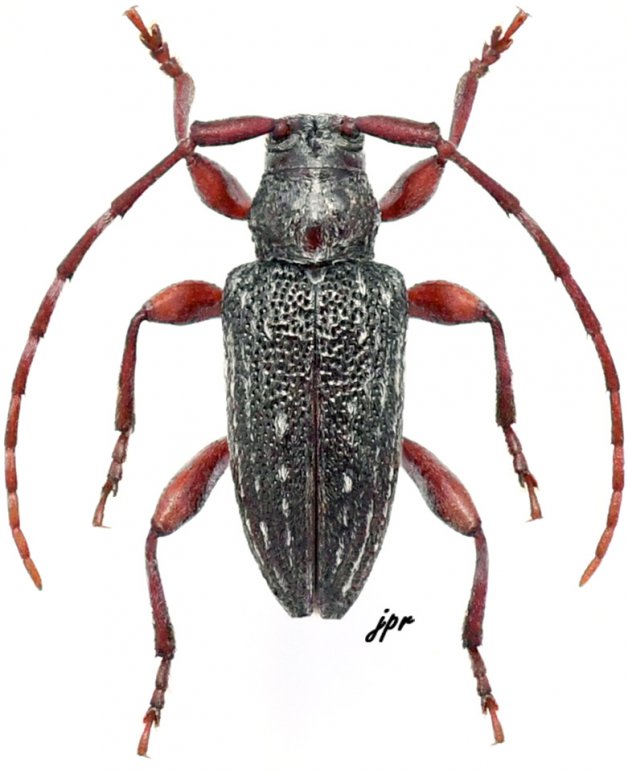This image features a detailed top-down view of an insect resembling a beetle set against a white background. The beetle’s body is mainly black with white specks, displaying a textured, pockmarked appearance. It has six legs, divided into three pairs: the front pair extending forward, the middle pair positioned downwards, and the back pair also directed downwards. Each leg is predominantly red, thick at the upper segments (thighs) and narrowing towards the ends with fine extensions.

The insect has two long, backward-curving antennas that almost form a semicircle around its body, running the entire length of its frame. It also features red eyes. In the bottom right corner, between the beetle's hind legs and its rear, there are black, cursive lowercase letters "jpr."